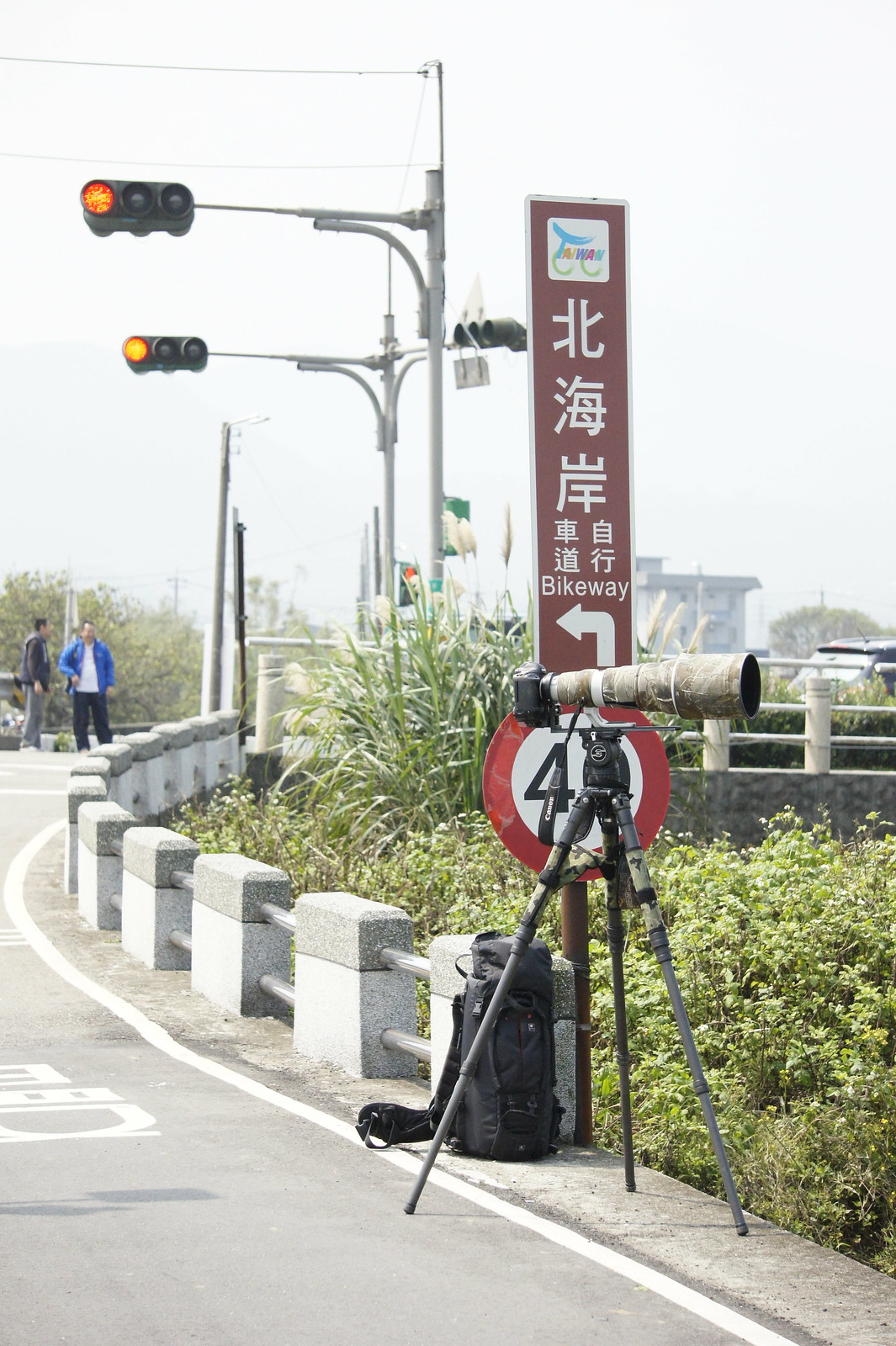This detailed photograph, taken in portrait mode on a sunny day, captures a curving cement roadway edged with a white stripe that meanders into the distance and curves off to the right. On the left side of the image, there is a road bordered by fencing, while to the right, a notable telescope with a long lens stands atop a tripod at the roadside. At the base of the tripod rests a black canvas backpack, presumably holding additional components for the telescope setup.

Adjacent to this equipment is a rectangular brown sign with Asian characters, likely Japanese or Chinese, and the word "bikeway" at the bottom with a white arrow directing left. Nearby, another traffic sign displays a 40 km/h speed limit within a red circle. Further into the background, two horizontally oriented traffic lights feature red signals on the leftmost light of each fixture.

The image also includes two men standing near the top of the road, one dressed in a dark grey jacket with light grey pants, and the other in a blue shirt or jacket over a white t-shirt with dark grey or black pants. Surrounding the area, scattered patches of vegetation, including pampas grass with green stems and yellow-white inflorescences, flutter into view. In the distant background on the right, a grey building with a flat roof and a rectangular structure on top peeks through additional, somewhat blurry foliage, completing this vibrant and bustling roadside scene.